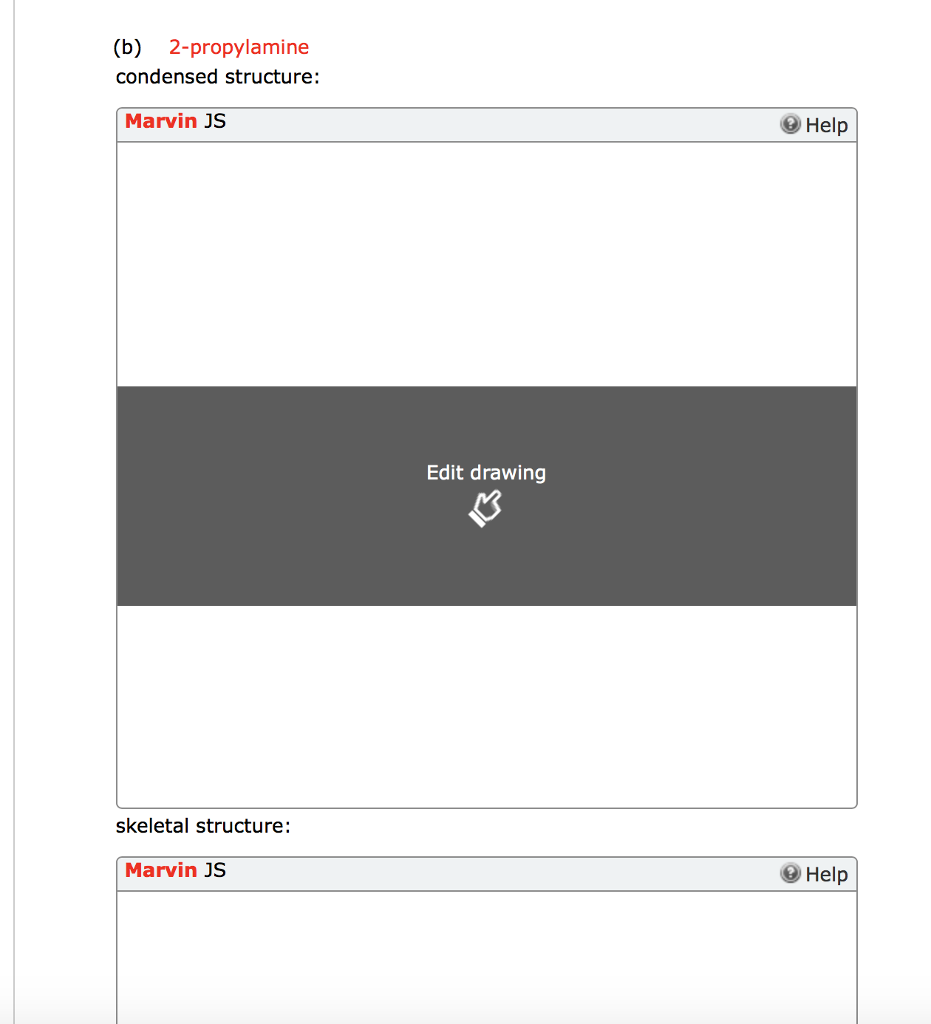The vertically rectangular image features a predominantly white background with two boxes stacked atop each other. The focal point begins outside and above the top box where there is a lowercase 'b' enclosed in parentheses situated in the upper left corner. Adjacent to this, written in red, is the term "2-propylamine." 

Directly beneath this in black text is the phrase "condensed structure." Within the top box, the upper left corner displays the word "Marvin" in red, followed by "JS" in black. The majority of this box remains white, barring a dark gray horizontal banner across the center, embossed with "Edit Drawing" in white lettering. 

Below this, in the space between the upper and lower boxes, the words "Skeletal Structure" are inscribed on the left side in black text. The lower box is partially visible, showing its top section. Similar to the first box, the upper left corner of this box reads "Marvin" in red, followed by "JS" in black.